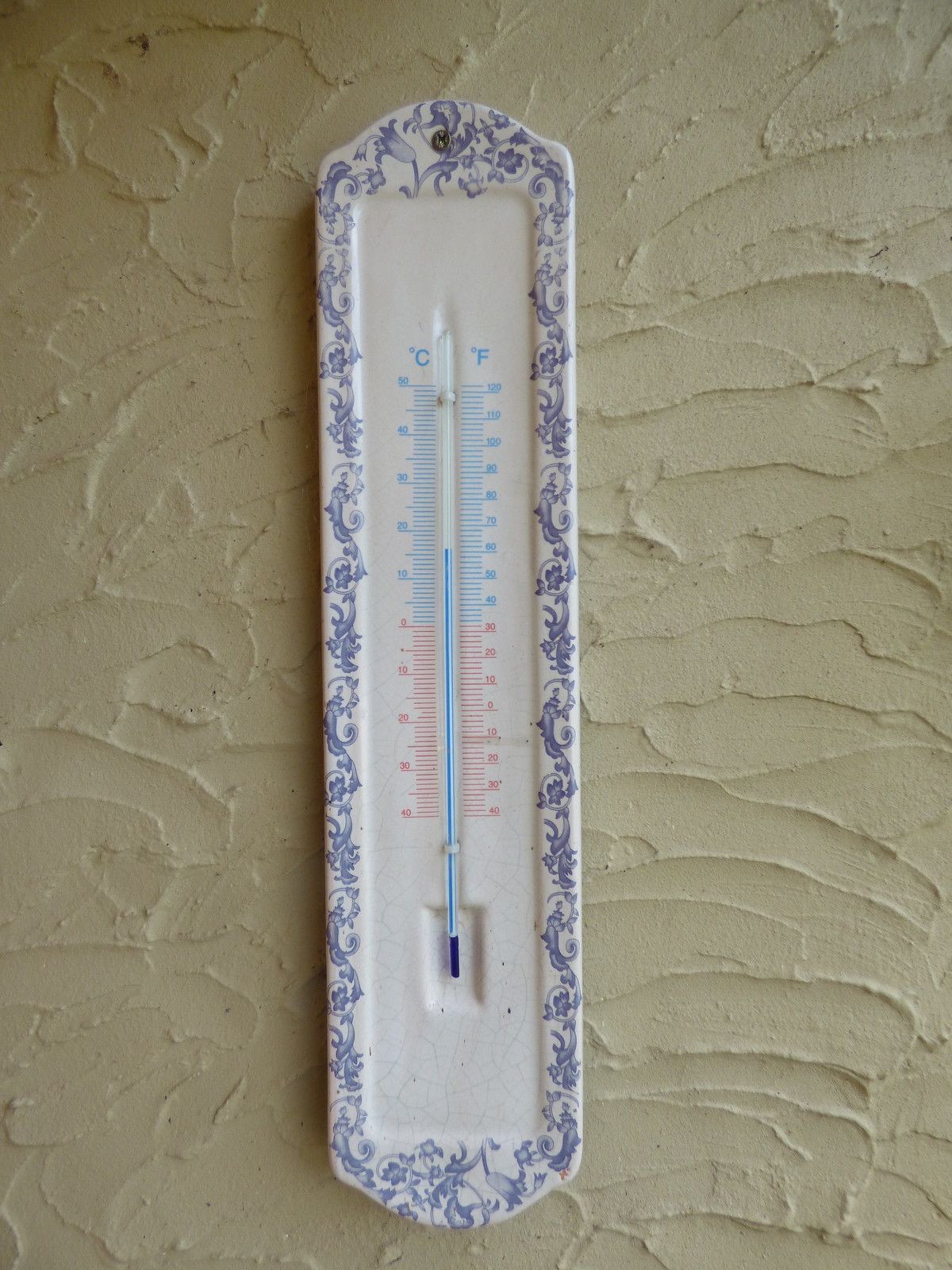This color photograph captures a thickly painted white wall, prominently displaying a vintage mercury thermometer at its center. The thermometer is encased in a decorative white frame adorned with an ornate blue floral design that encircles its cover. A small screw at the top affixes the thermometer securely to the wall. The device features dual temperature scales: Celsius on the left, displaying approximately 16 degrees, and Fahrenheit on the right, showing about 60 degrees. This carefully composed image excludes any people, writing, animals, plants, flowers, or signs, highlighting the stark contrast between the intricate design of the thermometer and the plain, textured surface of the wall.